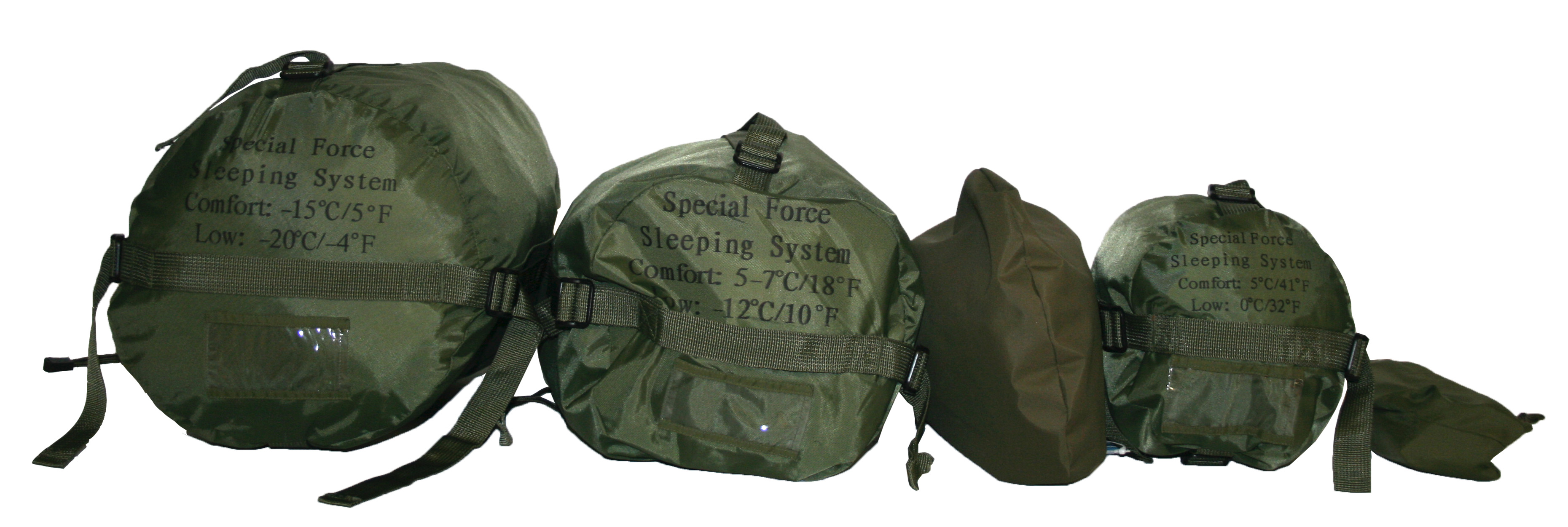The image depicts a lineup of four military-green bags, resembling various-shaped backpacks or duffle bags, likely designed for army purposes. They are arranged from left to right, varying in size, with the largest on the left and the smallest on the right. Each bag is labeled "Special Forces Sleeping System," with inscriptions indicating different comfort and temperature ratings. The largest bag is rated for comfort at -15 degrees Celsius (5 degrees Fahrenheit) and can endure lows of -20 degrees Celsius (-4 degrees Fahrenheit). The smaller bags also display temperature ratings, though less extreme, with the smallest rating not visible in the image. All the bags feature buckles and straps, reinforcing their rugged military design. Three of the bags are a uniform military green, while the smallest bag is a slightly different shade and is partially obscured, making its details difficult to discern.